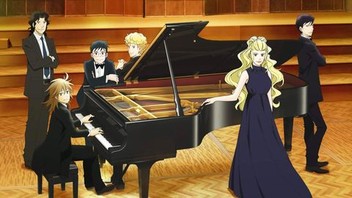In this detailed anime-style illustration, a grand black piano is the central focus, standing majestically on a light-patterned wooden floor. The backdrop is an elegant stage adorned with light brown and golden steps. Surrounding the piano are six characters, all dressed in formal attire. To the right, a man in a black suit casually leans against the piano, while a woman with long blonde hair, wearing a black gown that gracefully trails on the floor, rests her hand on the piano beside him. To the left, a man with longer blonde hair, dressed in a suit, sits poised on the piano bench, ready to play. Behind him, three more men in black suits or tuxedos complete the ensemble, creating a sophisticated and harmonious setting. The overall scene exudes a sense of anticipation and elegance, capturing a moment of poised readiness before a grand performance.